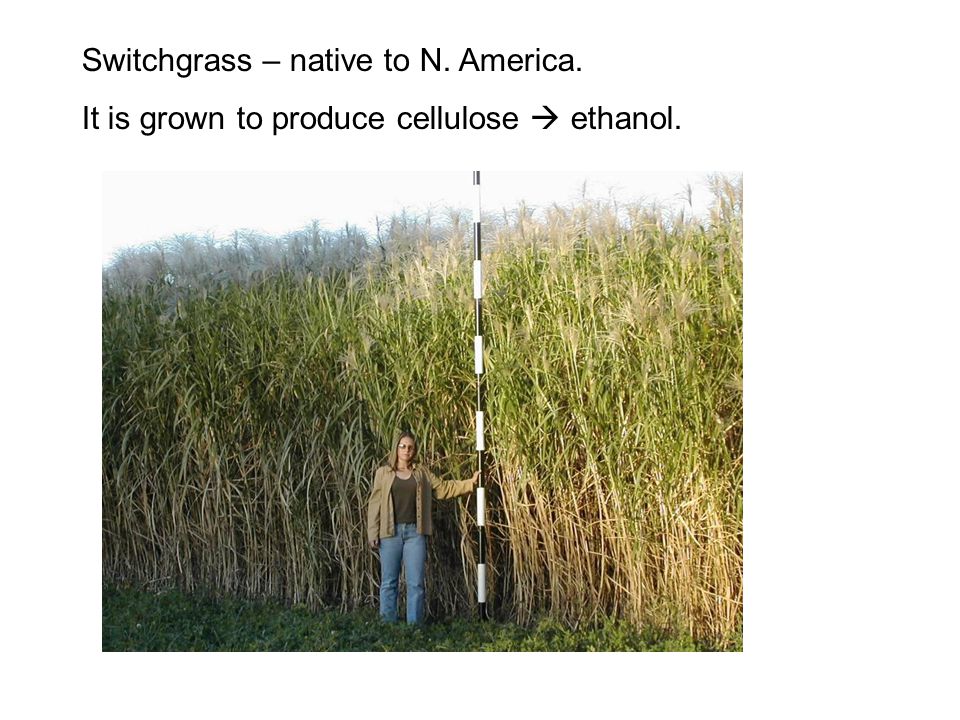This outdoor photograph features a woman standing amidst very tall switchgrass, which dominates the background and is about twice her height. The switchgrass, noted for its application in producing cellulose-ethanol, has brown stems at the base that transition to green midway up and end in brown feathery tips. The woman, positioned centrally and facing the camera, is wearing blue jeans, a brown jacket with a dark undershirt, and glasses. Her straight, shoulder-length dark blonde hair is visible. She stands on short grass in the foreground while holding a tall pole with alternating thick black and white stripes in her left hand. Above the image, text in black font reads: "Switchgrass native to N America. It is grown to produce cellulose-ethanol." The pole extends well beyond her height, reaching the top of the image, further emphasizing the scale of the grass behind her.